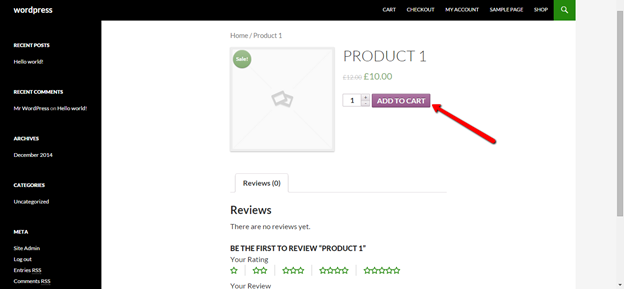This screenshot from WordPress features an e-commerce page for "Product 1." A prominent red arrow highlights the "ADD TO CART" button, which is presented in bold, purple text with all capital letters. Adjacent to it is a numerical input box allowing users to select the quantity of the product they wish to purchase, with the default value set to 1. To the right of these elements is a blank placeholder image labeled "Product 1," which is priced at £10. The section below indicates that the product currently has zero reviews and invites users to "Be the first to review Product 1." An adjacent star rating system offers options ranging from 1 to 5 stars for customer ratings.